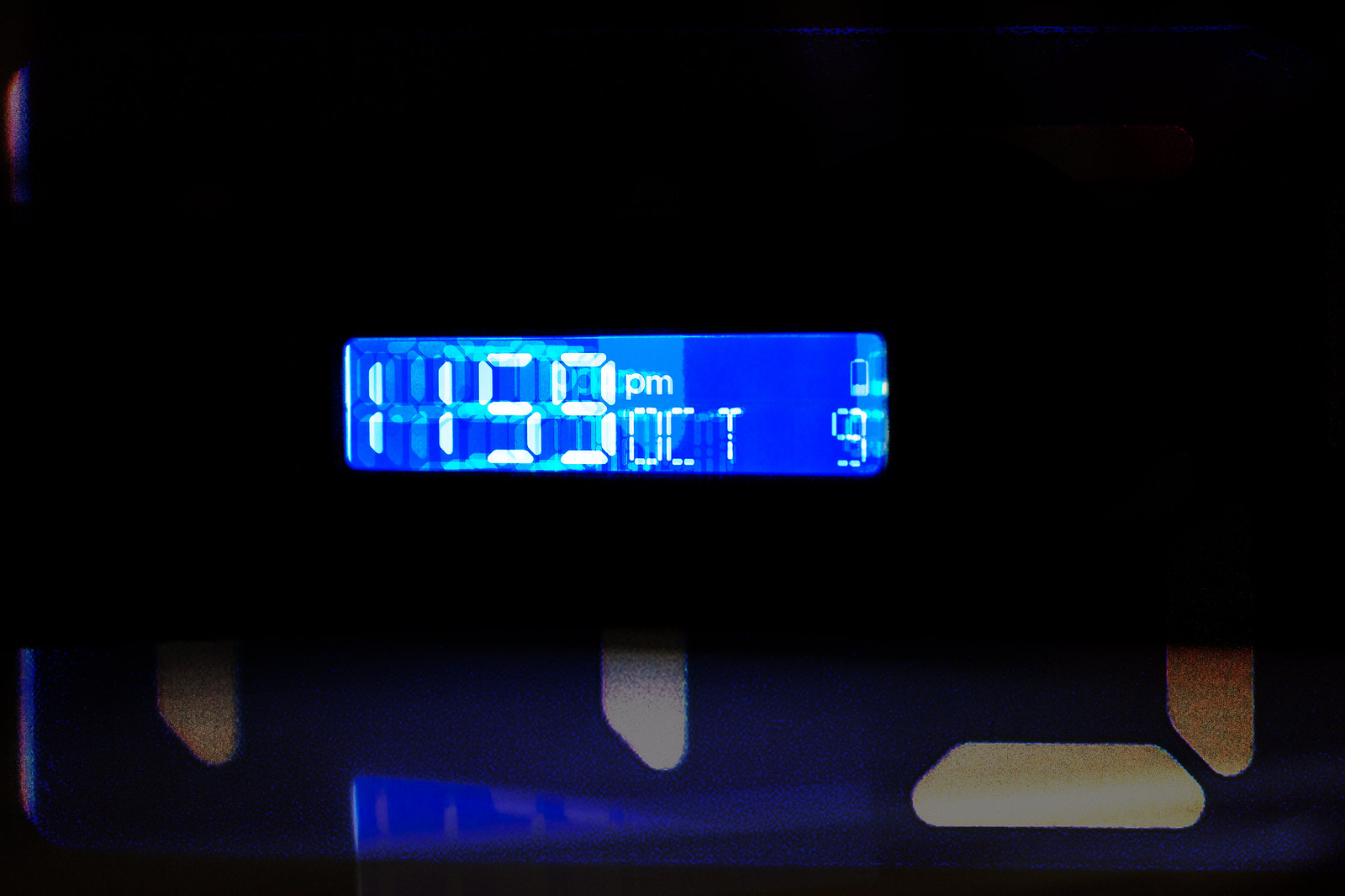A predominantly black image features a large rectangular digital display at the center. The lower portion of the image is covered in a deep black shade, gradually blending into the partially visible strokes of an unidentifiable digital number, lending an enigmatic fade-in effect. Dominating the center is a vivid blue digital readout with varying shades of blue, ranging from deep royal blue to lighter tones. It prominently shows "11:59 p.m." in bold, sizable text, followed by "October 9th" in a much thinner and narrower font style. The entire display appears somewhat blurry, adding to the overall mystique of the image against its stark black background.